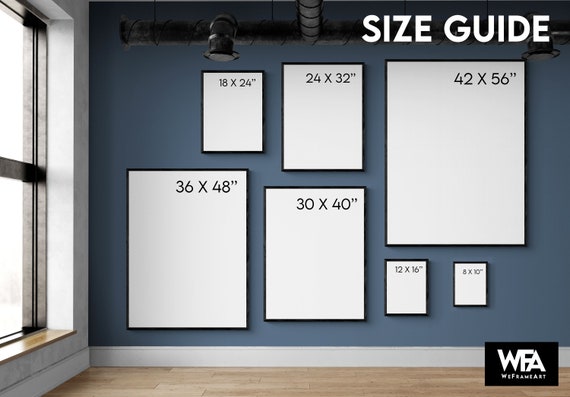This image features a spacious room with a dark navy blue wall as the backdrop. There is a window on the left-hand side, casting natural light. Centered on the wall, a collection of variously sized white-framed photographs are displayed, each frame marked with dimensions such as 8x10 inches, 12x16 inches, 18x24 inches, 24x32 inches, 30x40 inches, 36x48 inches, and 42x56 inches. The frames are arranged in a visually appealing manner to serve as a size comparison chart. At the top right-hand corner, bold white text reads "Size Guide," providing a reference for potential buyers to gauge the size of photographs or artworks for their space. In the bottom right-hand corner, the company logo, "WFA - We Frame Art," is clearly visible. This horizontal image functions as a detailed visual aid, helping customers make informed decisions about their frame size options.